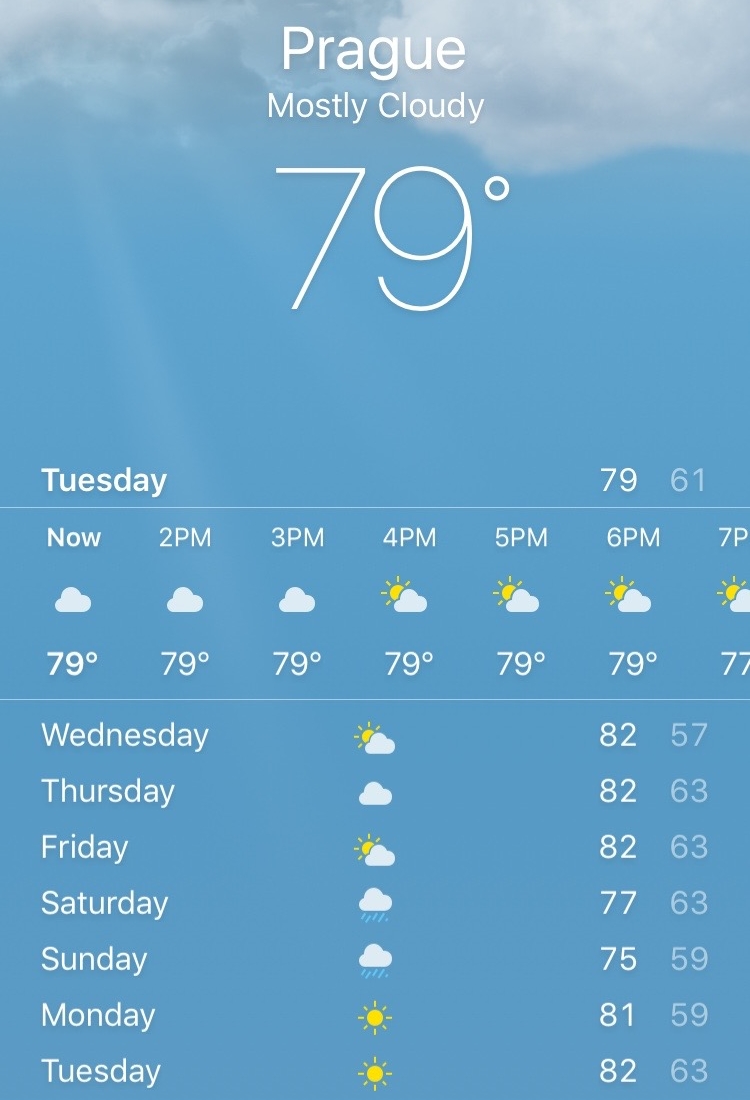Vertical screenshot of a weather application for the city of Prague, displaying a bright blue sky background with clouds and sun rays peeking through. The current weather conditions indicate it is mostly cloudy with a temperature of 79°F, likely Fahrenheit given the context. The hourly forecast for Tuesday shows a consistent temperature of 79°F from 2 p.m. through 6 p.m., dropping slightly to 77°F by 7 p.m.

The weekly outlook is as follows:
- **Wednesday**: High of 82°F, low of 57°F, mostly cloudy.
- **Thursday**: High of 82°F, low of 63°F, partly cloudy.
- **Friday**: High of 82°F, low of 63°F, mostly sunny.
- **Saturday**: High of 77°F, low of 63°F, rain expected.
- **Sunday**: High of 75°F, low of 59°F, rain expected.
- **Monday**: High of 81°F, low of 59°F, mostly sunny.
- **Tuesday**: High of 82°F, low of 63°F, partly cloudy.

The app clearly outlines daily highs and lows along with varying weather conditions, from mostly cloudy and partly cloudy days to periods of rain over the weekend.